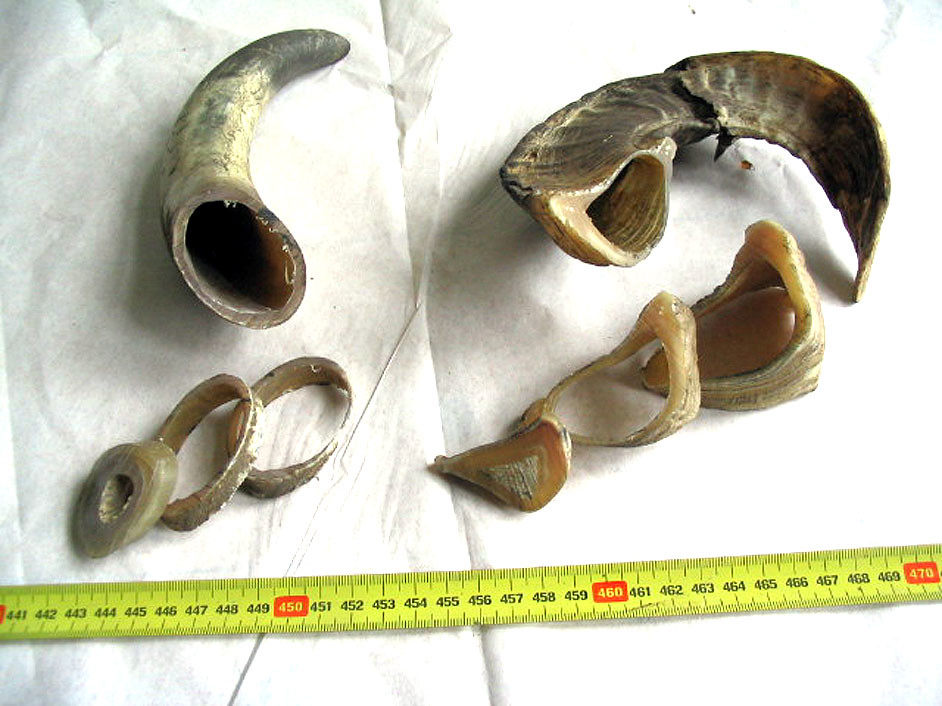This indoor color close-up photograph displays a collection of animal horns and bones arranged on a white cloth or paper background. To the left of center, there is a tan horn with a dark brown tip, curved to the right and hollow on the inside. Below this horn are several slices of what appears to be the same horn, each about half an inch thick. These slices are stacked, showcasing their brown, uncleaned surfaces. To the right, there is a broader ram's horn, shaped like an upside-down "U" and also hollow in the center. Accompanying this are more horn slices, similar in thickness to those on the left, with some having small knobs or irregular circular shapes reflective of the internal structure of the horn. At the bottom of the photograph, a yellow tape measure is visible, with measurements in millimeters ranging from 450 to 470. The overall scene is well-lit, with light coming from the right, casting slight shadows to the left. The entire image is free of any text or printing, allowing full focus on the natural textures and details of the horns and bones.